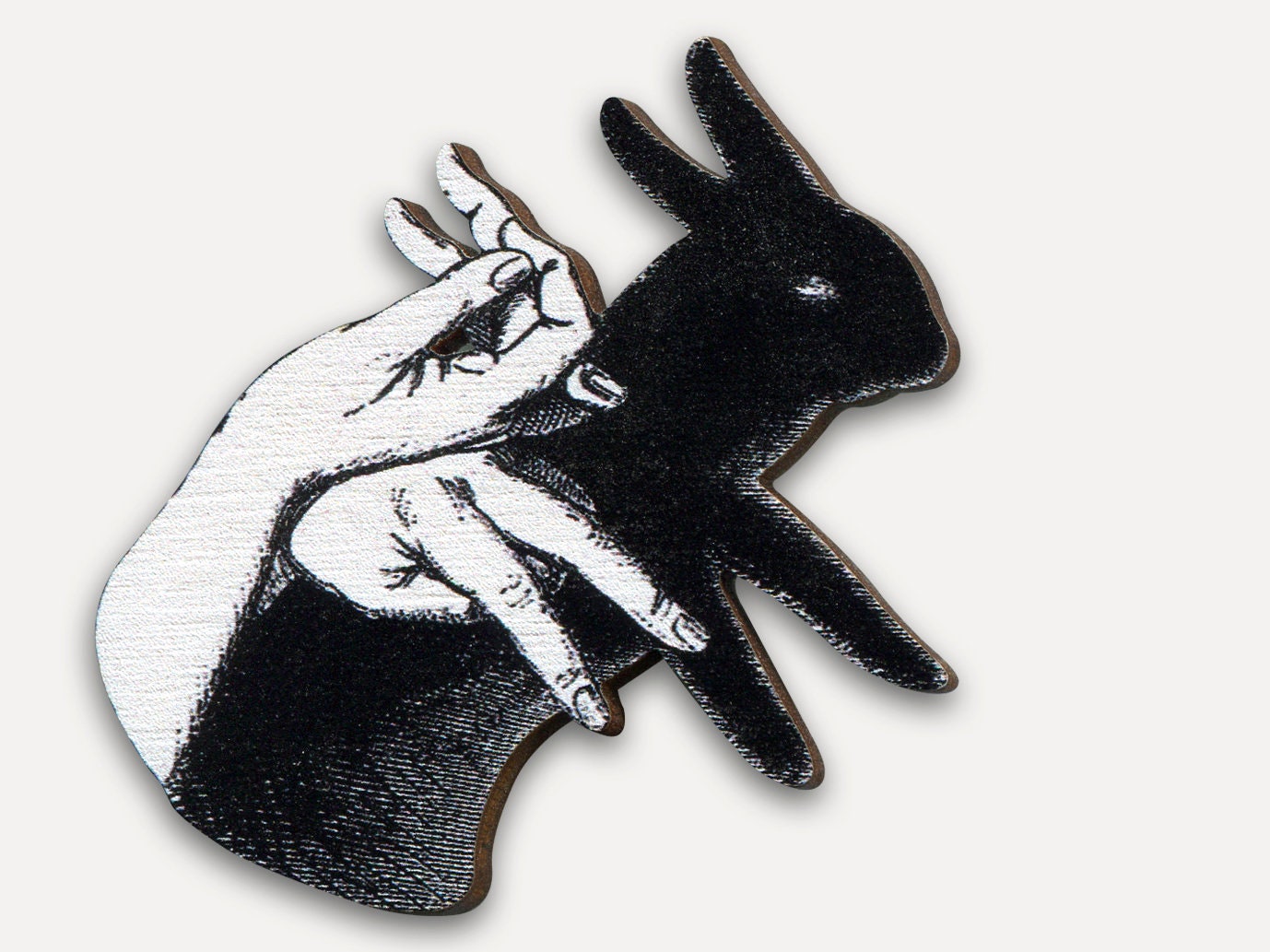The artwork is a detailed wood carving displayed on a white surface or wall. It prominently features the black silhouette of a rabbit, positioned slightly right of center with its head pointing to the right. The rabbit's ears extend towards the top left, while its arms stretch in a zigzag fashion towards the bottom right. Overlaying the rabbit's form are the shadows of two hands, capturing the essence of a shadow puppet. These hands, emerging from the bottom left, are carefully arranged to mimic the rabbit's features—one hand forms the rabbit's head with its thumb and fingers pinched together, and the other imitates the rabbit's arms with its fingers extended outward. The intricate interplay between the carved rabbit and the shadow hands evokes the whimsical practice of creating shadow animals on a wall.